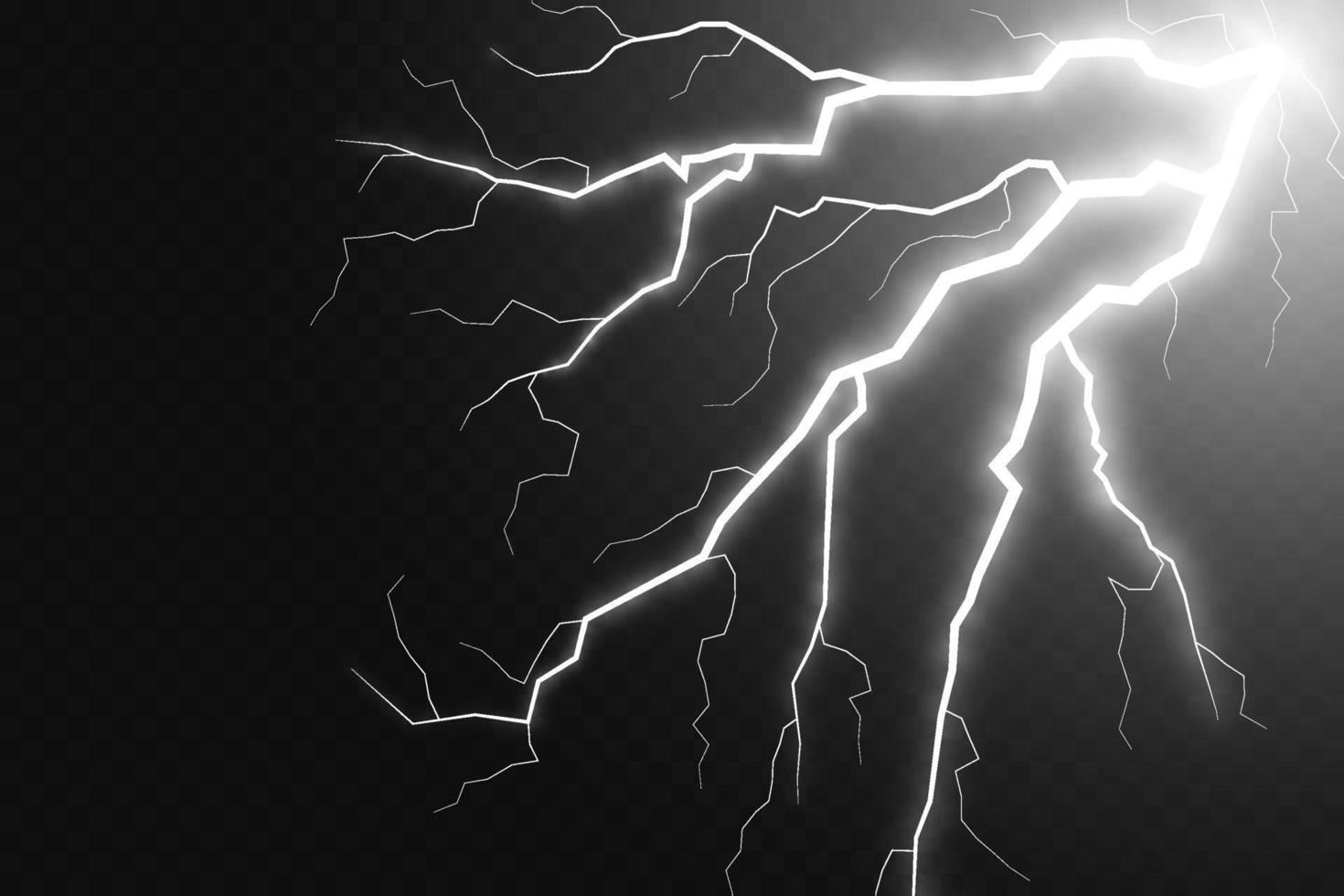This detailed image appears to be a computer-generated illustration of lightning striking across a gradient background. The lightning originates from the upper right-hand corner of the image, extending diagonally to the bottom left corner. The lightning bolt is white and starts off brighter at its origin, gradually becoming less bright as it stretches out. It features three main shafts, with numerous smaller bolts branching off each one. The backdrop is a black and dark gray checkerboard pattern that fades from lighter near the lightning's origin to darker towards the bottom left. This gradient enhances the contrast, making the lightning stand out vividly against the pixelated background.